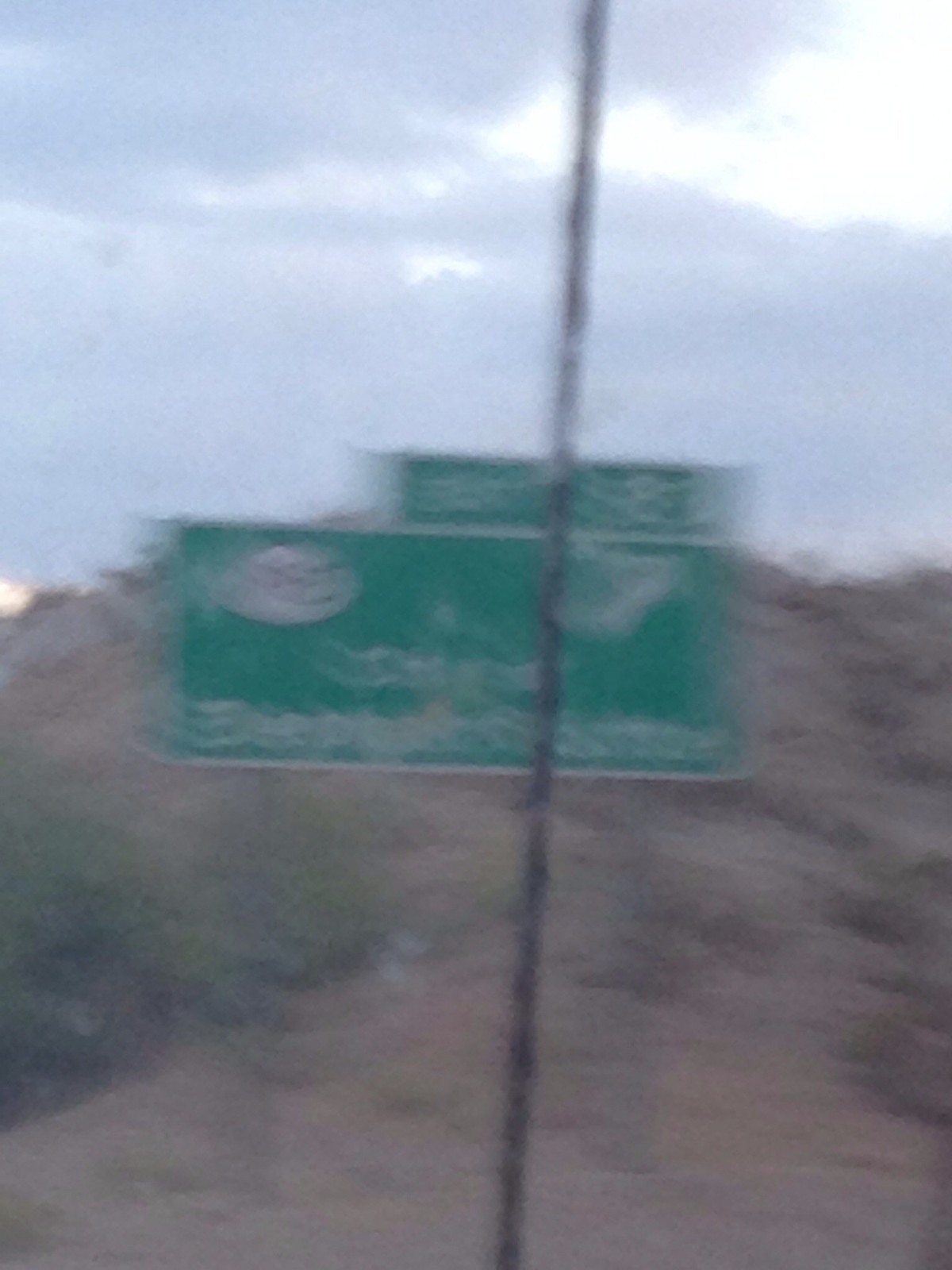This is a very blurry color photograph taken outdoors, depicting a green road sign on a brown hillside. The green sign is situated below the top third of the image, with a cloudy gray and white sky dominating the upper portion. The sign, which has an unreadable white oval in the upper left-hand corner and more white writing across its center and bottom edge, also features a smaller rectangular green sign on its right side, also bearing white text.

The hill behind the sign is primarily composed of dark brown earth with sparse patches of green and brown grass, as well as some rocks. Ill-defined due to the photograph's poor focus, the sky includes gray clouds with a hint of light peeking through in the upper right-hand corner. The overall scene is viewed from a low angle, looking upward toward the sign and into the sky.